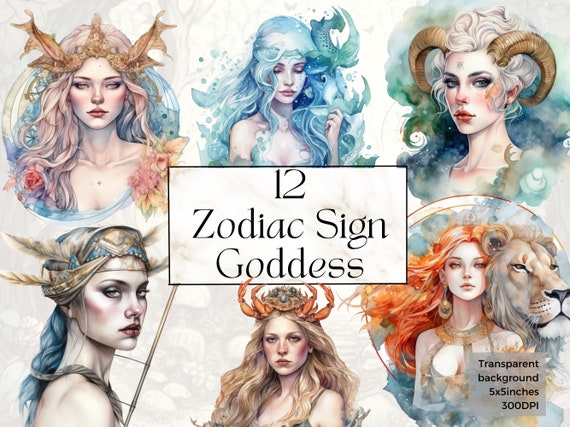The image is an artistic representation (likely a digital painting or colored pencil drawing) titled "12 Zodiac Sign Goddesses," divided into six sections arranged in two rows of three. Each section features a woman depicted from the mid-chest upward. The top left portrays a woman with pink hair adorned with a crown of leaves, surrounded by blue swirls and flowers on her right. The central top section showcases a woman with blue hair, eyes closed, and surrounded by fish. The top right features a woman with white hair styled in a bun, goat horns, and green and blue swirls around her. In the bottom left, there's a woman with blue hair in a ponytail, feathers in her hair, a crown, and a rope going across her chest. The central bottom section shows a woman with blonde hair and crab legs protruding from her head. Lastly, the bottom right displays a woman with reddish-orange hair standing beside a tiger. The text "transparent background, 5 by 5 inches, 300 dpi, deep penetration" is noted in the bottom right corner of the image.